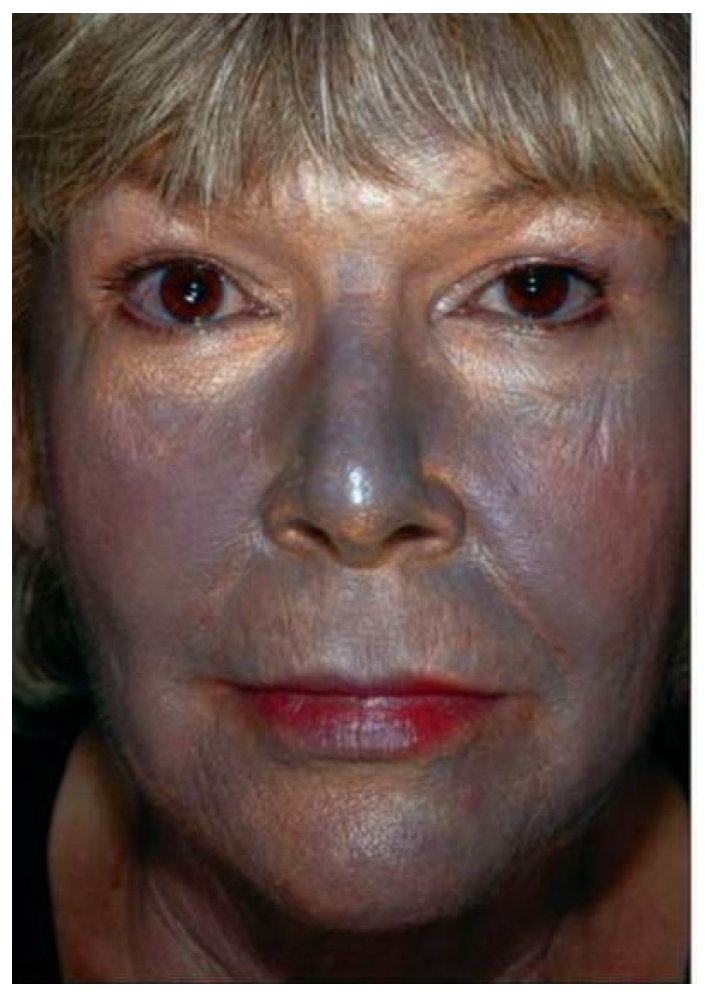This indoor color photograph features an extreme close-up of a Caucasian woman’s face, which completely fills the frame, revealing a detailed and intricate portrayal. At approximately 45 to 50 years old, she has striking brown eyes that gaze directly at the camera with a gentle expression. She sports blonde bangs that hang down to just above her eyebrows, partially concealing them. Her hairline is visible, but the top of her head is cropped out. Her complexion shows a dramatic contrast of colors and texture; her face appears to be adorned with stage makeup, possibly for a costume, with dark grayish tones accentuating her features. There are also vivid purples and pinks around her cheekbones, nose, and the lower half of her face, suggesting further artistic makeup rather than natural pigmentation. Her lips are painted a bold red, and she has a thin upper lip contrasted by a fuller lower lip. She is dressed in a black cotton shirt, and only a small portion of her neck and ear is visible. The rectangular photo emphasizes her face, capturing every detail with precision.